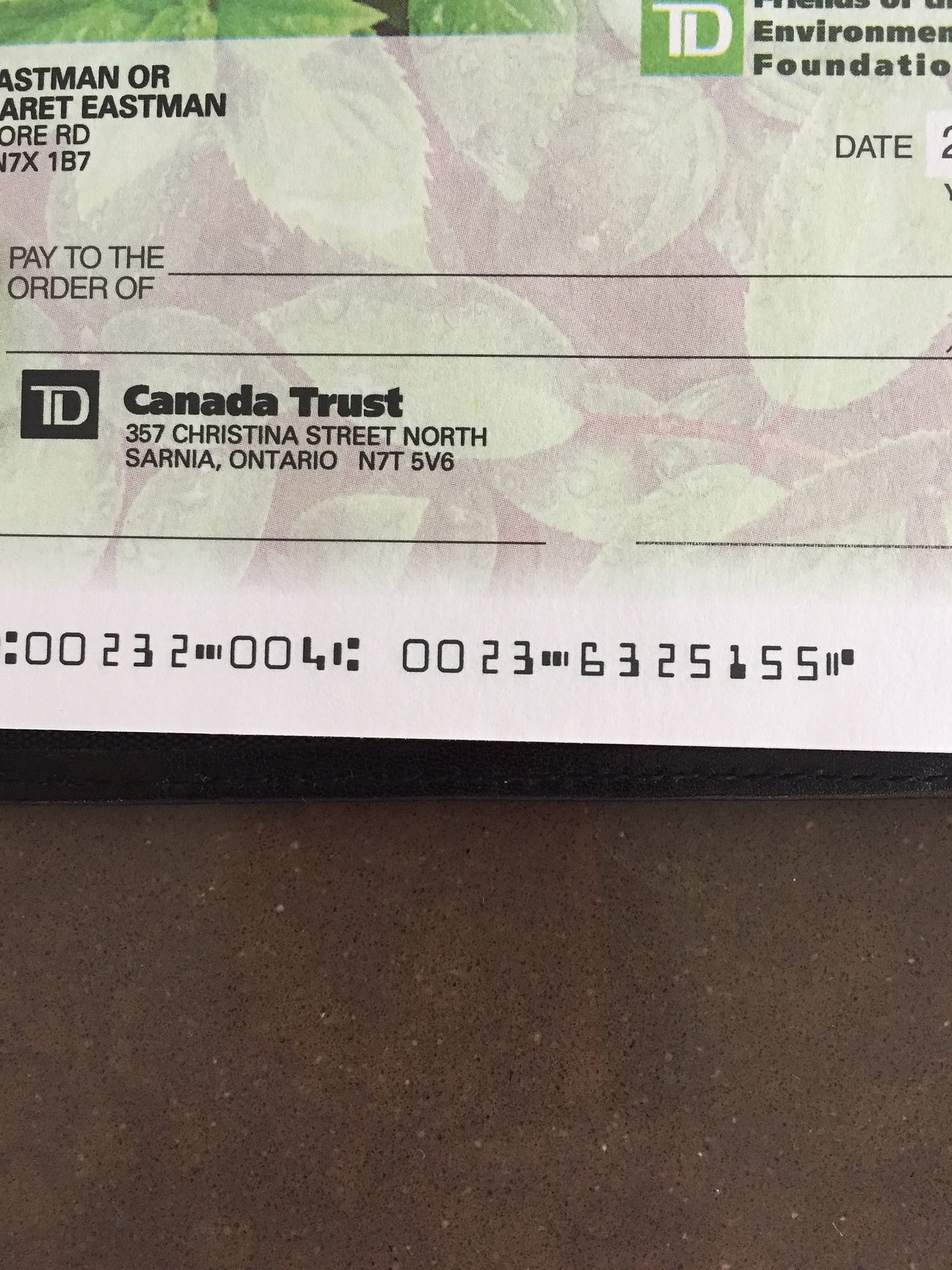The photograph depicts a partially cropped, unfilled check from TD Bank, set against a backdrop that resembles a brown, dusty surface. The check itself is predominantly white with a transparent background of green tea leaves behind the text. In the upper left corner, the name "Eastman" is visible, suggesting the issuer. On the right-hand side, a green square with the white letters "TD" indicates the bank logo. Adjacent to the logo, partially visible text reads "environment foundation." The check features a section for the date, although only part of the number "2" is visible. The text "pay to the order of" remains unfilled. At the bottom, the check shows the black text "Canada Trust 357 Christina Street North, Sarnia, Ontario N75V6," accompanied by serial numbers "0023200" and "00236325155." The overall appearance of the check, including the faded leaf imagery and multiple fields left blank, suggests it is ready for personalization.